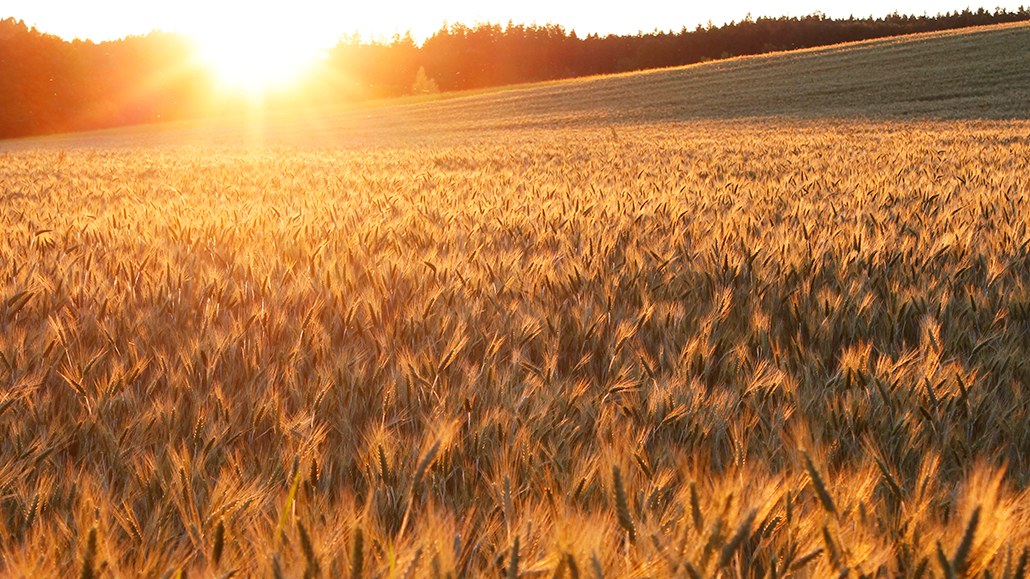A breathtaking landscape showcases a golden field of wheat stretched across rolling hills. In the foreground, individual stalks of wheat shimmer under the intense radiance of the sun, creating an almost sparkling effect. The scene bathes in the warm, glowing orange hues of a setting sun, whose glaring light is so intense that it almost feels painful. The sun itself appears as a massive ball of light in the top left, casting rays that radiate throughout the image and illuminate the wheat, making it look almost golden. There's a play of light and shadow as the hills slope upwards toward the background, where a large shadow extends down the slope, contrasting with the illuminated grains in the foreground. Far off in the distance, the silhouette of a tree line creates the illusion of distant mountains, adding depth to the scene. Though individual plants in the shaded areas are indistinct, the movement of the wheat in the wind is almost palpable, creating an immersive feeling that transports you to this serene, farm-like setting at dusk.